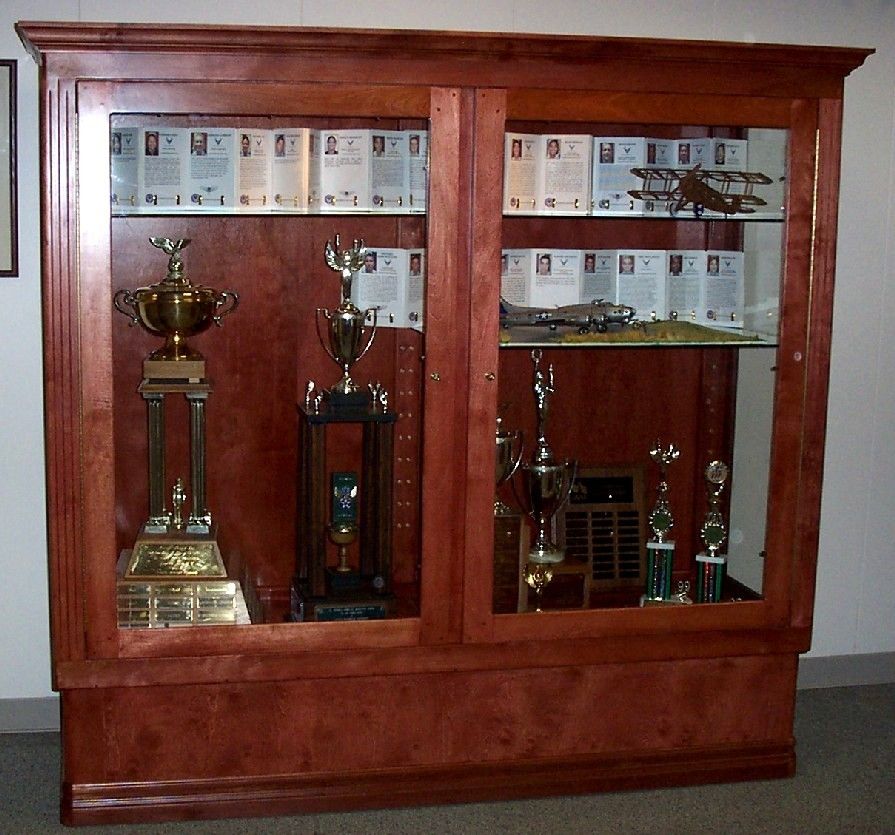The image showcases a prominently placed rectangular display cabinet made of shiny, reddish-tarnished mahogany wood with glass doors, standing against a white concrete wall on a gray floor. The cabinet features multiple shelves: on the bottom shelf, there are six trophies, with two tall ones on the left and four shorter ones on the right. The upper shelves contain various items, including two old-style airplane models marked with a U.S. Air Force logo. Adjacent to these models are several photographs with descriptions, depicting people who presumably received awards related to aircraft activities. The upper shelf also displays additional pictures that provide biographical details of these individuals. The whole arrangement reflects a history of achievements in aviation, meticulously presented within the confines of this polished wooden display.